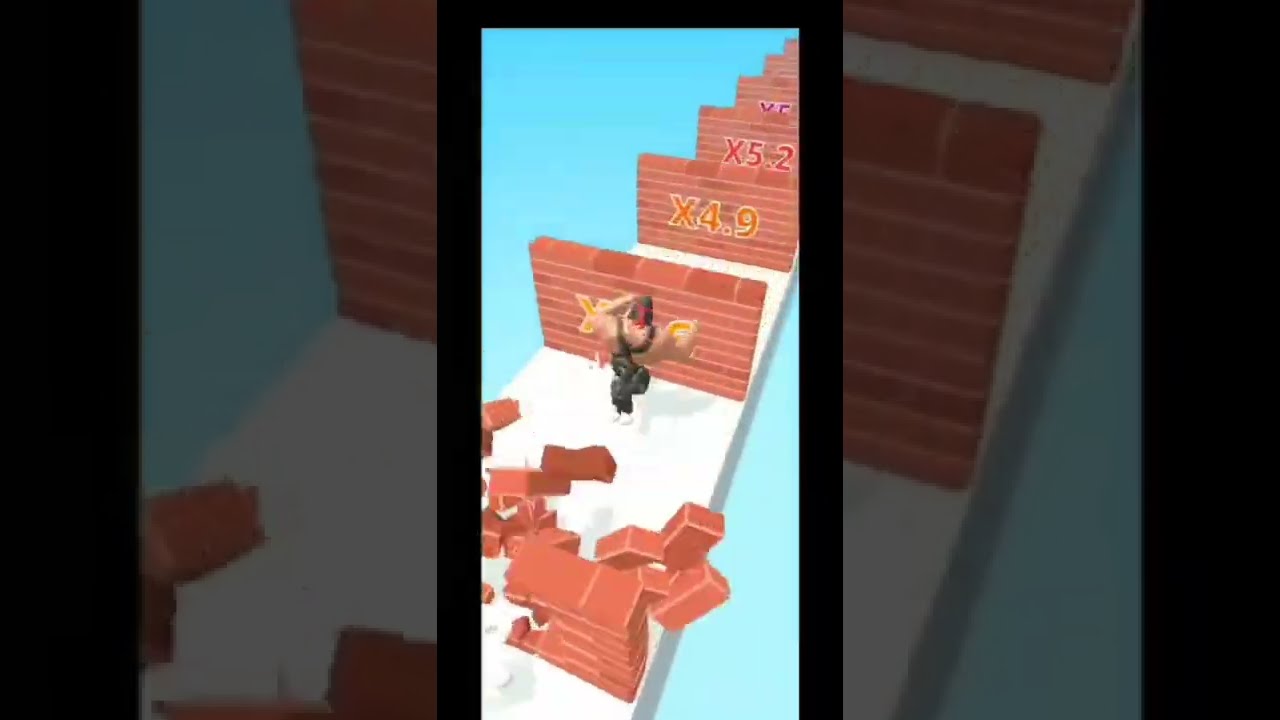The image is a vertical screenshot from a video game, framed by a black border. A central, narrow rectangular section displays a muscular figure, possibly styled after Rambo, wearing a green tank top, camo pants, white shoes, and a red bandana tied around brown hair. He appears to be breaking through a series of brick walls on a raised white walkway. The wall he is currently breaking has writing on it, and behind it are more brick walls marked with "X 4.9" in orange and "X 5.2" in red. The figure has already shattered a brick wall behind him, leaving crumbled remnants. The background is blue, presumably representing sky or water. To the left and right of the central image are blurred, zoomed-in sections of the same scene, showing detailed portions of the walls and the platform the character is on.